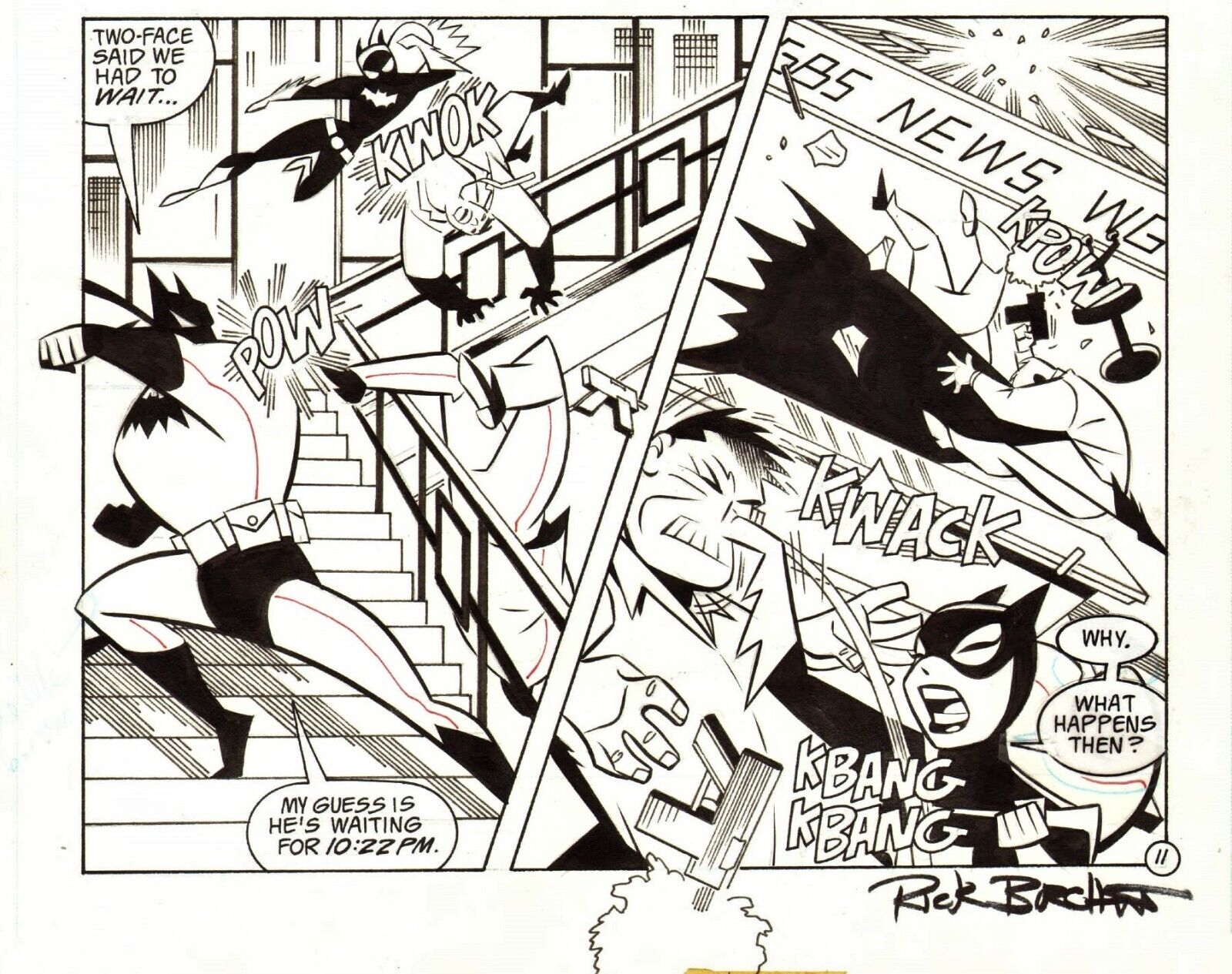This black-and-white comic panel, reminiscent of vintage newspaper comics, features Batman and Batgirl in a dynamic action sequence. The panel is split diagonally, with intense fight scenes on both sides. On the left, Batman stands on a staircase, remarking, "Two-Face said we had to wait," just before delivering a powerful punch to a bad guy, knocking him over a stair railing with an emphasized "Pow!" Batgirl, on the other hand, is engaged with a large mobster, disarming him of his submachine pistol with a punch that resounds with a "Quack" and "Bang Bang." Batgirl questions, "Why, what happens then?" Meanwhile, Batman speculates, "My guess is he's waiting for 10-22 PM." In the background, action words like "Kapow" and "Quack" highlight the frenetic energy. The artwork is signed by an artist named Rick, whose last name remains partially unclear.